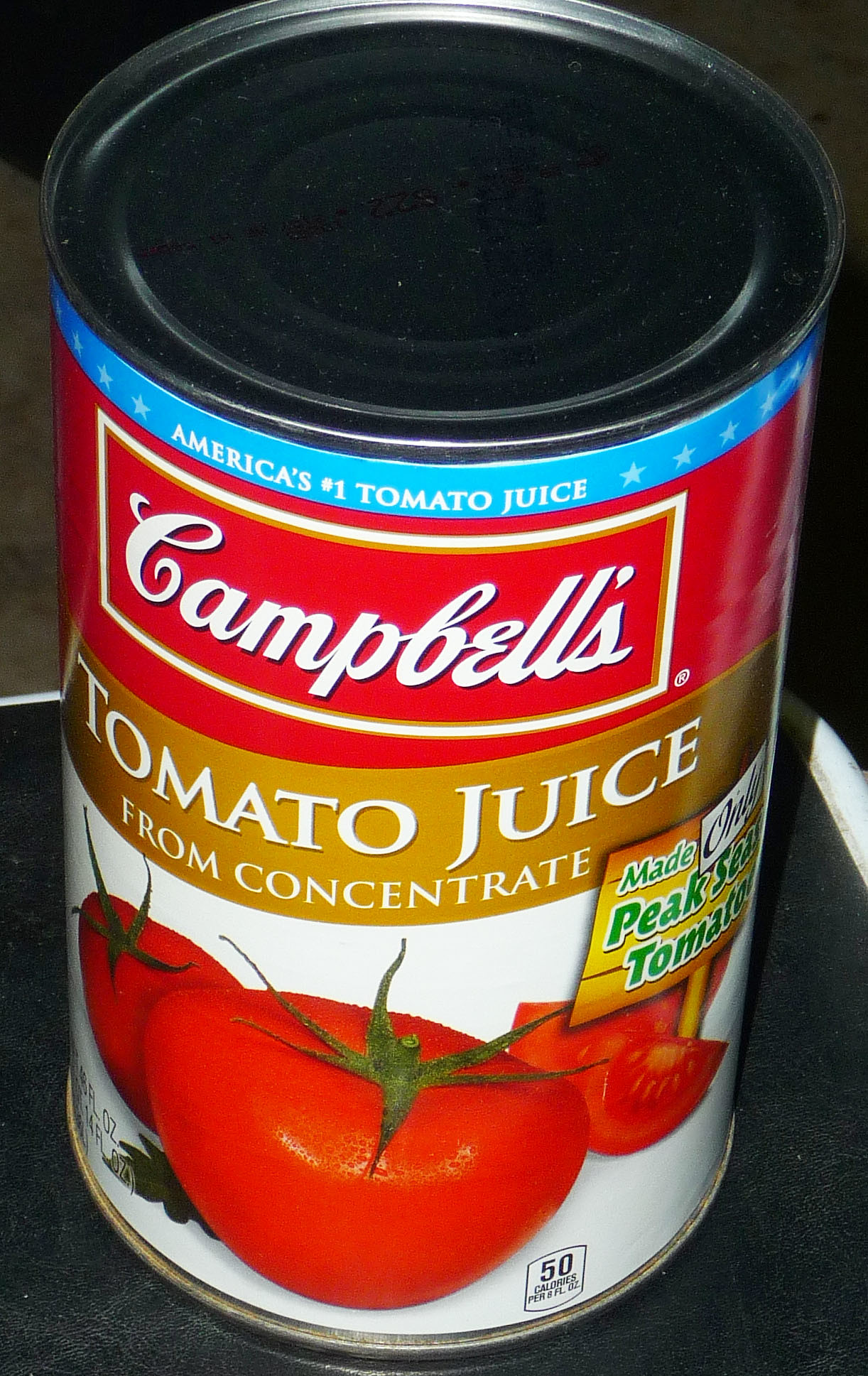This photograph captures a large cylindrical tin can of Campbell's Tomato Juice prominently displayed on a sleek black surface. The vibrant label on the can draws immediate attention: its upper half is a striking red, featuring the iconic Campbell's logo, while the bottom half transitions to a clean white backdrop adorned with vivid images of ripe red tomatoes, complete with green stems, and a succulent wedge of sliced tomato. A distinguished gold stripe accentuates the label, proudly declaring "Tomato Juice from Concentrate," and an additional inscription assures that the juice is "Made only from peak season tomatoes." This meticulously designed label not only reflects the premium quality of the product but also celebrates the freshness and rich flavor embodied in every can.